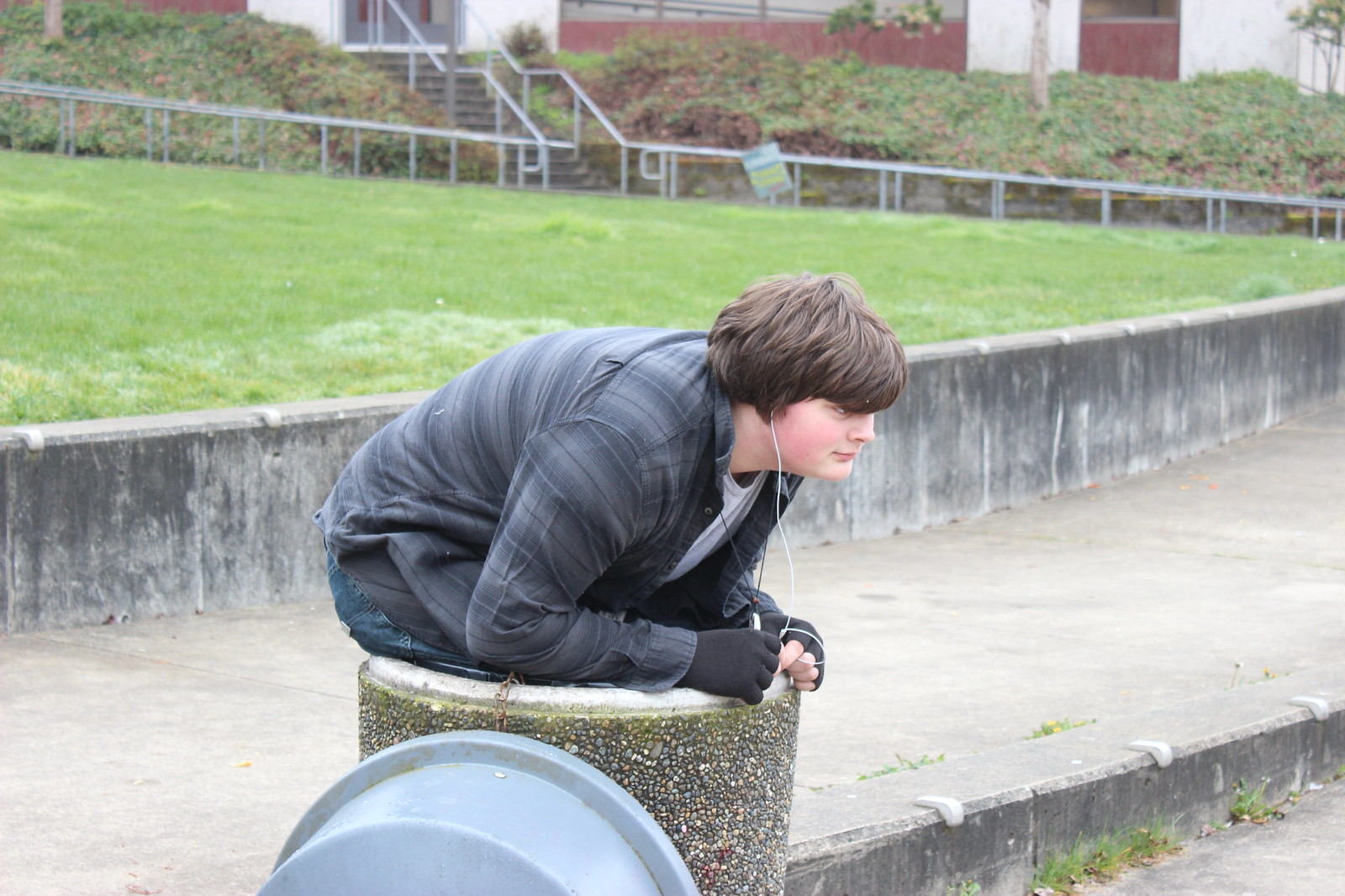In a color landscape photograph, a teenage boy with shaggy, dark brown hair sits intentionally inside a trash can, leaning against its stone-lined rim. The trash can's large, round, gray plastic lid, attached by a rusty metal chain, is propped up against the bin. The boy, approximately 13 years old, wears a gray and black striped hoodie with a white shirt underneath, blue jeans, and black fingerless gloves. Earbuds are snugly fitted in his ears. The trash can is positioned on a concrete sidewalk, which leads to a set of stairs with metal railings. Behind the boy is a small grassy area and a building, suggesting a school or similar structure. The composition falls under photographic representational realism, capturing a stark, realistic depiction of the scene.